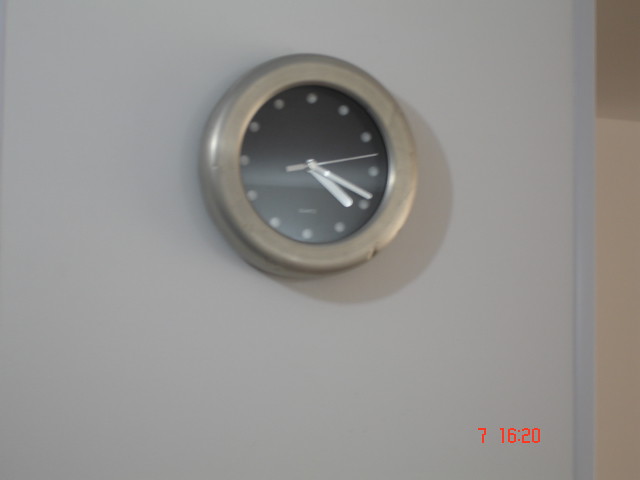In the image, there is a visible timestamp at 7:16:20. The setting features a wall that transitions from white to beige. Mounted on this wall is a small, circular clock with a metal frame. The face of the clock is a dark gray, almost black, color. Instead of numbers, the clock features twelve gray circles marking the hours. Both the hands—including the hour, minute, and second hands—are also gray. The clock shows the time as 4:18.